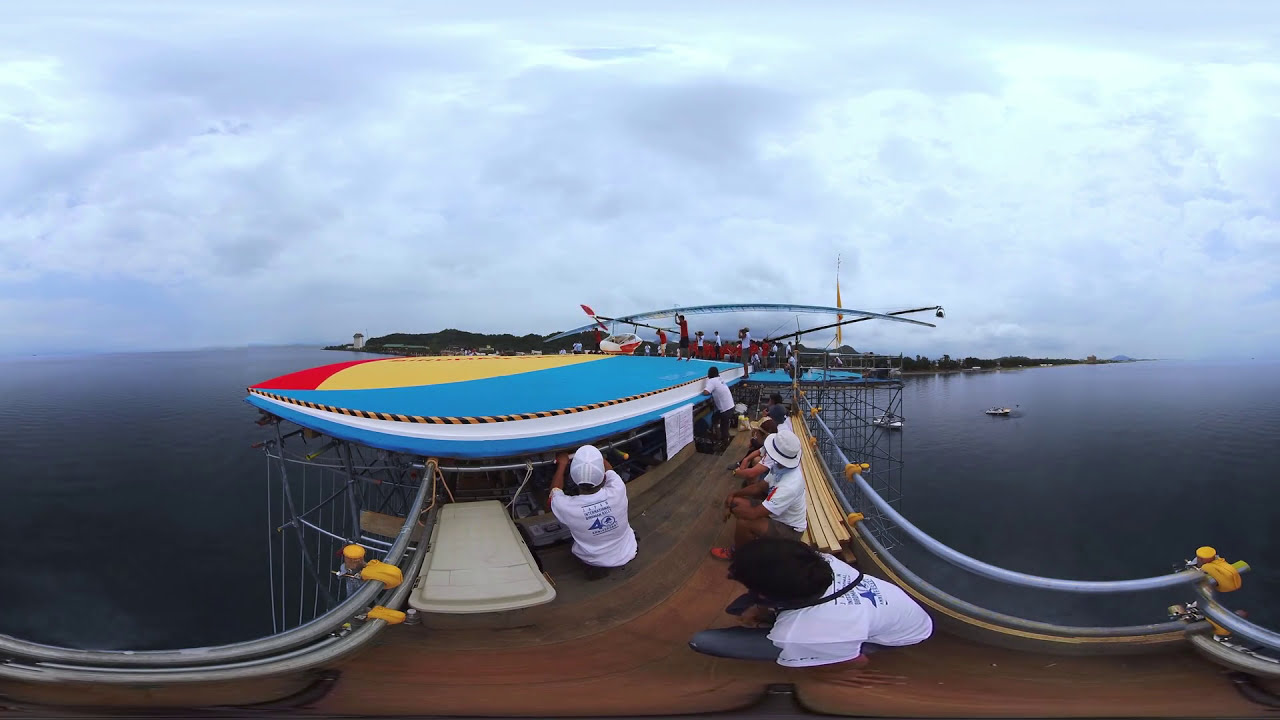The image depicts a bustling scene on a dock surrounded by an expanse of ocean. At the center, a large metallic platform adorned with a multicolored blue, yellow, and red tarp stands out, resembling a parachute. Seated along the platform's edge on wooden planks or logs are numerous individuals, some in white shirts with logos and blue writing, others in red shirts. They appear engaged in assembling something, possibly a glider or related project, hinting at a collaborative effort. Metal railings encircle this area, and a caution barrier with yellow and black stripes adds to the organized yet industrious atmosphere. In the background, additional people can be seen against the backdrop of boats in the water and distant land dotted with trees and potential residential zones. Overhead, a gray, cloudy sky looms, casting a somber tone on the otherwise industrious scene. A white and red aircraft, either a helicopter or a plane, also features in the image, adding to the sense of large-scale activity.